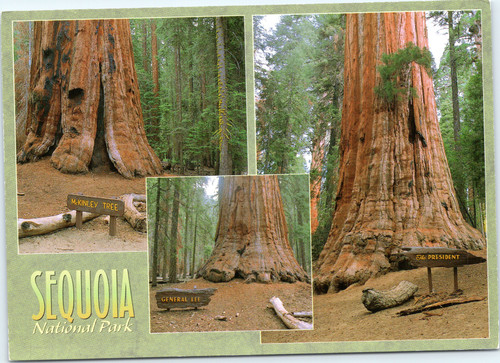This collage-themed postcard features three iconic photographs of giant trees from Sequoia National Park, framed by a dark green border. In the bottom left corner, gradient yellow-to-green text reads "Sequoia," followed by "National Park" beneath in yellow text. The top left photograph showcases the massive "McKinley Tree," standing tall with a log and a wooden sign bearing its name in yellow font in the foreground. Behind this tree, a dense forest of smaller fir and pine trees extends into the background. The center photograph, the smallest and stacked above the others, features another imposing tree labeled "General Lee" on a similar wooden sign with yellow text. This tree also stands amidst a lush, green forest. The final photograph on the right captures yet another grand tree, marked by the sign "The President" in yellow text, with branches adorned with green vegetation and another log at its base. The rich, reddish-brown hue of the trees stands out against the verdant backdrop, creating a striking visual representation of Sequoia National Park's natural beauty.